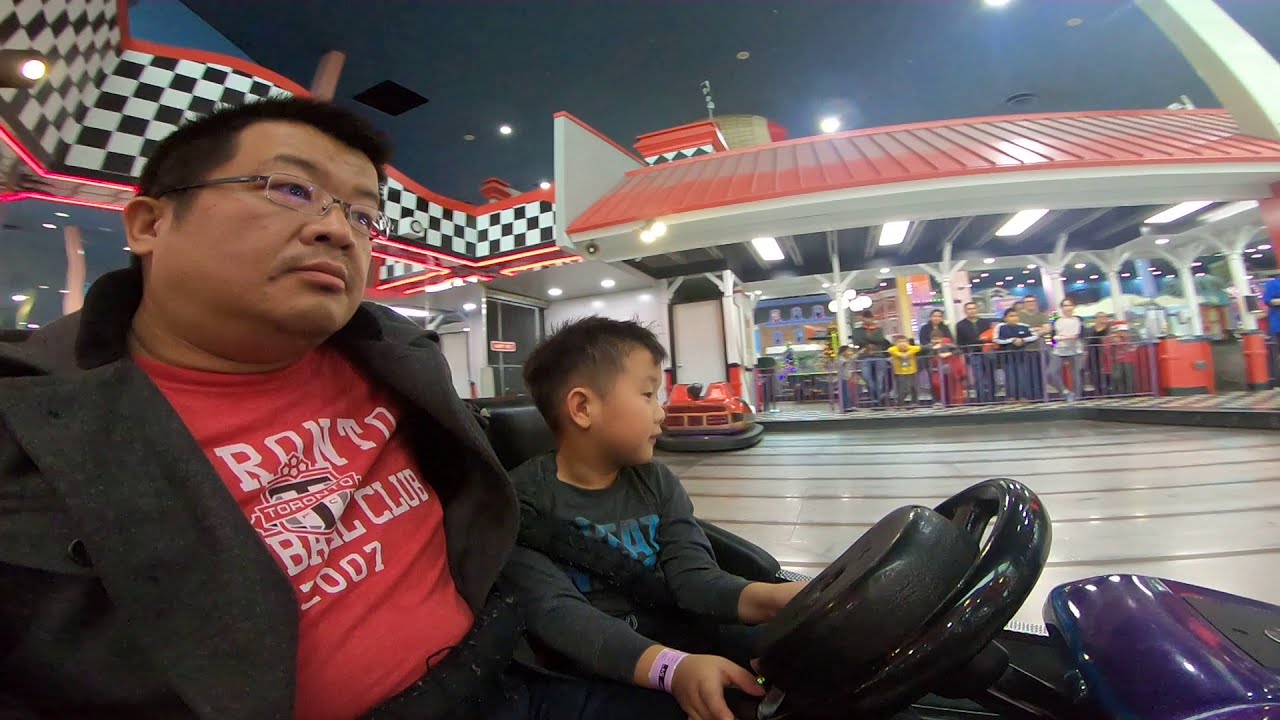The photograph captures a detailed scene of an Asian man and a young boy, possibly his son, riding in a dark blue or purple go-kart at an outdoor track. The man, who appears to be in his late 30s or early 40s with short black hair and glasses, is wearing a black coat over a red shirt that reads "Toronto Ball Club 2007." He has a round, chubby face and sits on the left side of the image. The boy, around five or six years old, is dressed in a long-sleeve dark gray shirt with blue lettering and a white bracelet on his hand. He is positioned to the left of the man, with his hand gripping the shiny black steering wheel of the go-kart.

The background features a red-roofed building with a black and white checkered pattern along the front, enhancing the lively atmosphere of the go-kart track. Standing behind a railing, blurred out in the distance, are people likely waiting for their turn to ride. The scene appears to be set at night, as indicated by the black sky and hanging lights illuminating the area. To the right within the frame, part of a red bumper car is also visible, adding to the playful and vibrant mood of the photograph.